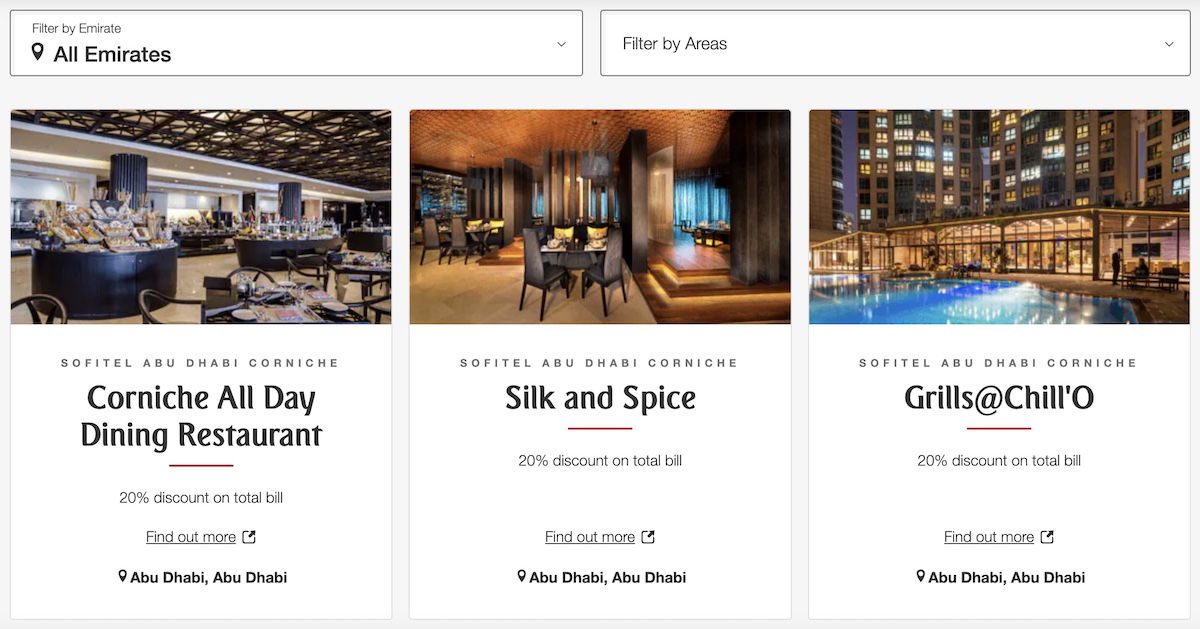The page features three prominent images against a primarily white background, accompanied by black text. At the top of the page, there are two clickable filter boxes: the first, located in the upper left, is labeled "Filter by Emirate" and includes all emirates. To its right, there's a box labeled "Filter by Area".

Beneath these filters are three main images, each portraying different restaurants within the Sofitel Abu Dhabi Corniche.

1. **First Image**: Depicts an elegant all-day dining restaurant at the Sofitel Abu Dhabi Corniche. The text highlights a 20% discount on the total bill and includes a prompt to "Find out more". The image is captioned with "Sofitel Abu Dhabi Corniche, Corniche All-Day Dining Restaurant, 20% discount on total bill, Abu Dhabi, Abu Dhabi".

2. **Second Image**: Shows another restaurant within the Sofitel Abu Dhabi Corniche, identified as "Silk and Spice". This image also advertises a 20% discount on the total bill and offers more information via a clickable link. The accompanying text reads "Sofitel Abu Dhabi Corniche, Silk and Spice, 20% discount on total bill, Abu Dhabi, Abu Dhabi".

3. **Third Image**: This photo appears to be taken from an exterior view, showing a poolside scene. It represents yet another dining option at the Sofitel Abu Dhabi Corniche, known as "Grills at Shillow". Similar to the others, it also offers a 20% discount on the total bill and includes a prompt to learn more. The text indicates "Sofitel Abu Dhabi Corniche, Grills at Shillow, 20% discount on total bill, Abu Dhabi, Abu Dhabi".

Overall, the webpage seems to serve as a booking or promotional platform for various dining experiences at the Sofitel Abu Dhabi Corniche, featuring substantial discounts and detailed descriptions of each restaurant.